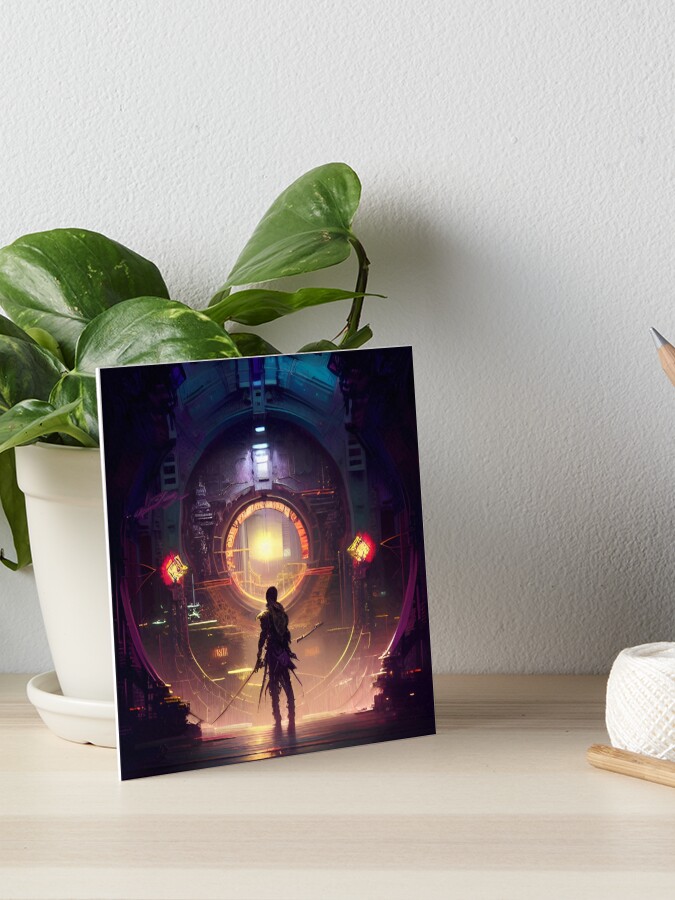In a cozy home decor setup, a striking unframed canvas is propped up against a vibrant green house plant in a white vase with a matching water catcher. The canvas, resting on a light beige wooden table, features a captivating science fiction scene. Dominated by dark shades of blue and black, with highlights of red, yellow, and purple, the image showcases a lone warrior-like figure standing in front of an impending locomotive or spaceship amidst a dark nighttime setting. Surrounding the setup, there is a silver pencil placed at the edge of the table and a ball of yarn nearby. The backdrop of the arrangement is a whitewashed wall, further enhancing the visual appeal of this intricate and imaginative display.